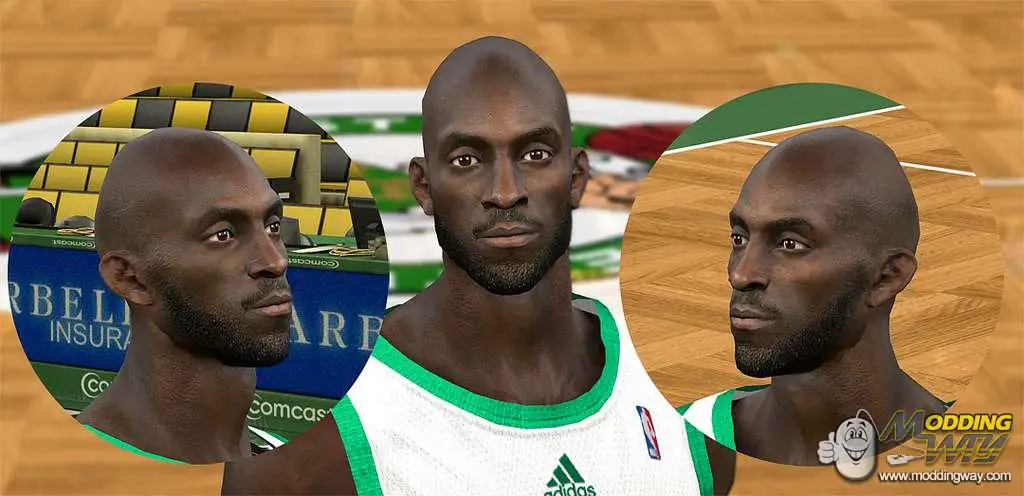The image prominently features a single individual, presumably a basketball player, standing on a basketball court marked with the Celtics logo at center court. The background displays bleachers, suggesting an indoor arena setting. The central figure is dressed in an Adidas basketball tank top and is facing slightly to the left while looking directly into the camera. Additionally, there are two circular overlays on the image: one on the left side showing the player's right profile, and one on the right side displaying the player's left profile, offering different angles of the same face.